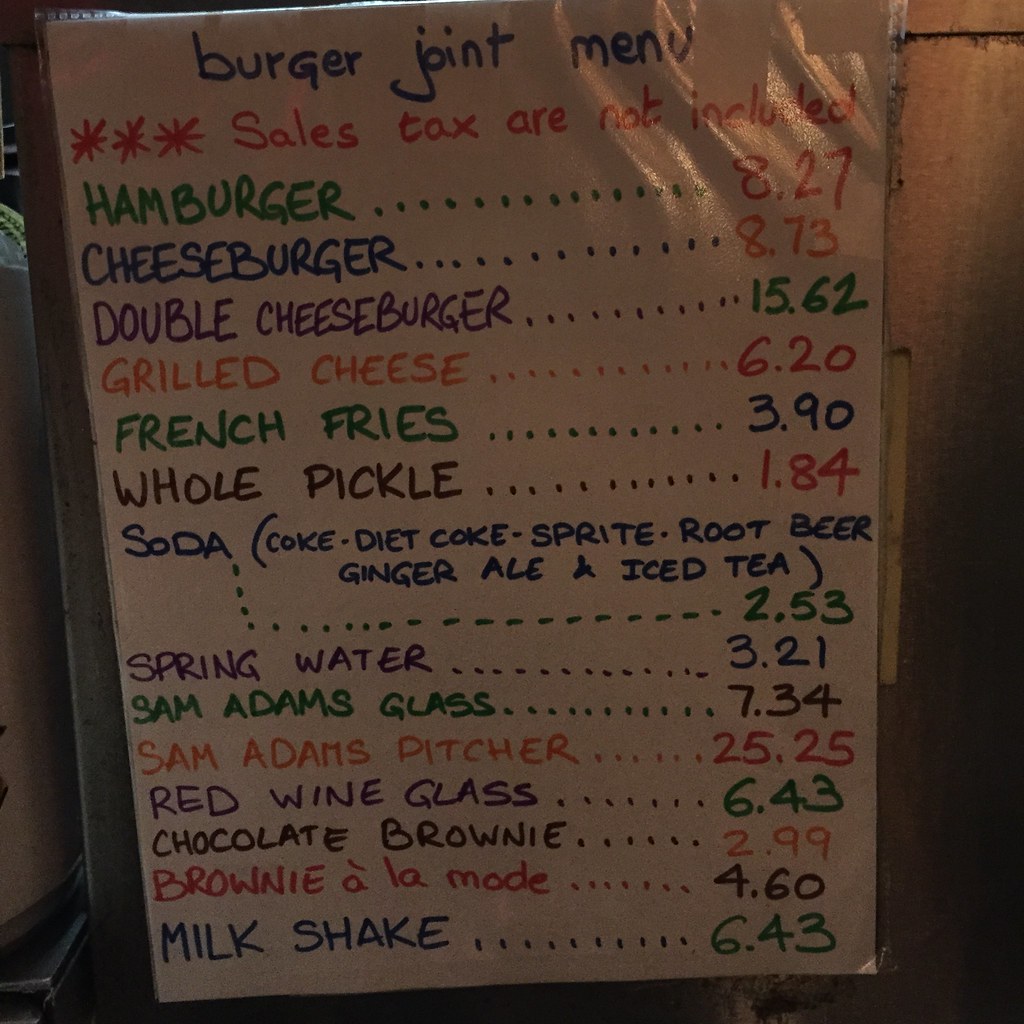The image depicts a gray-walled background featuring a prominently displayed menu encased in a white laminated sheet of paper. The menu is visually striking, with its text printed in alternating hues of blue, red, green, purple, and orange. At the top of the sheet, the title "Burger Joint Menu" is proudly displayed, followed by three asterisks and a disclaimer stating, "Sales tax are not included." 

Below the title, each menu item is meticulously listed, connected to its price by a series of dots. The offerings include:

- Hamburger ...... $8.27
- Cheeseburger ...... $8.73
- Double Cheeseburger ...... $15.62
- Grilled Cheese ...... $6.20
- French Fries ...... $3.90
- Whole Pickle ...... $1.84
- Soda (Coke, Diet Coke, Sprite, Root Beer, Ginger Ale, or Iced Tea) ...... $2.53
- Spring Water ...... $3.21
- Sam Adams (Glass) ...... $7.34
- Sam Adams (Pitcher) ...... $25.25
- Red Wine (Glass) ...... $6.43
- Chocolate Brownie ...... $2.99
- Brownie a la Mode ...... $4.60
- Milkshake ...... $6.43

The detailed and colorful presentation of the menu provides a cheerful and inviting glimpse into the dining options available at the establishment.